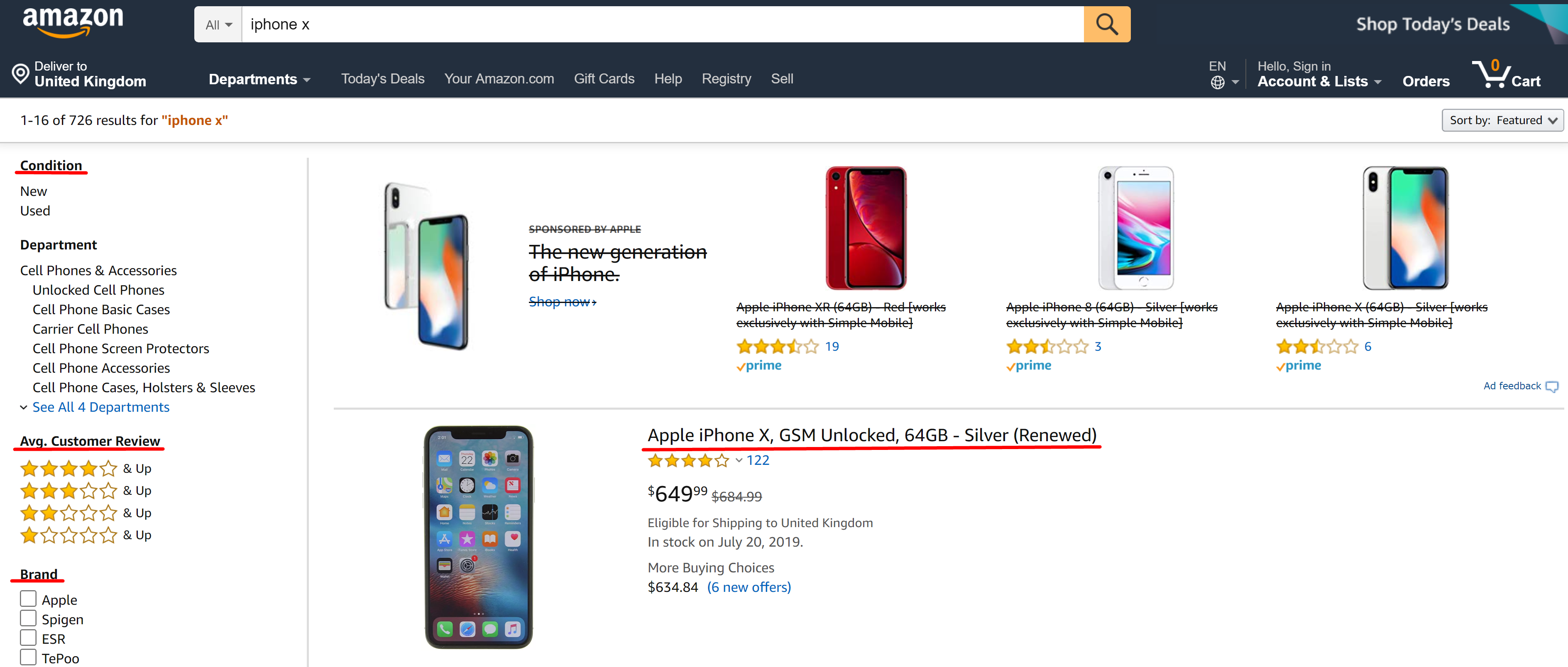The image showcases a webpage on Amazon, with the familiar Amazon logo displayed prominently on the top left corner, featuring an orange arrow that curves to the right. The search bar at the top contains the query "iPhone X," leading to a primary search result that features the "Apple iPhone X GSM Unlocked, 64GB, Silver (Renewed)" priced at $649.99. An image of the iPhone X accompanying the listing is also visible.

The navigation bar at the top offers various options such as "Delivered to United Kingdom," "Departments," "Today's Deals," "Your Amazon.com," "Gift Cards," "Help," "Registry," "Sell," as well as account-related options like "Hello, Sign in," "Accounts and Lists," and "Orders." Adjacent to these options is a cart icon.

On the left sidebar, there are numerous filtering options under different categories, including "Condition (New, Used)," "Departments (Cell Phones and Accessories, Unlocked Cell Phones, Basic Cases, Carrier Cell Phones, Cell Phone Screen Protectors, Cell Phone Accessories, Cell Phone Cases, Holsters and Sleeves)." Additionally, the page displays average customer reviews.

The search bar at the top also features a magnifying glass icon within an orange square, indicating the search function.